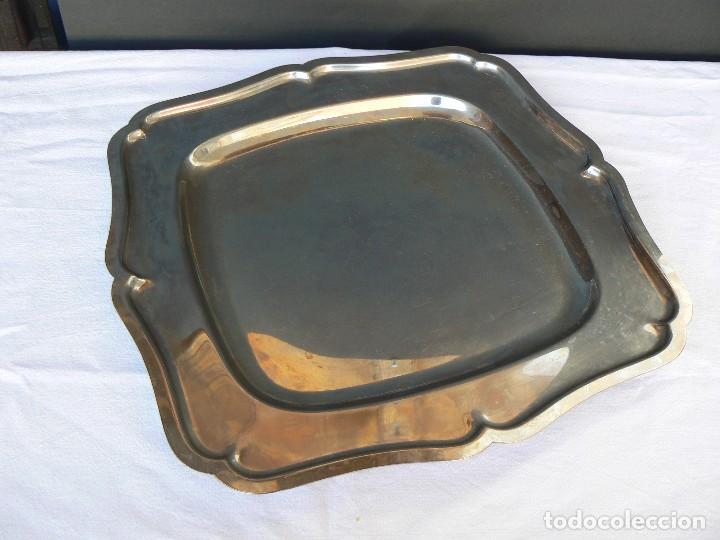The image depicts an old, rectangular silver serving platter with a distinct wear indicating its age. The platter is prominently centered on what appears to be a white tablecloth, occupying the majority of the white background. The serving platter features a curved edge with slight outward bends and pointed tips at the center of each side. Its surface, while once shiny, now shows signs of oxidation and grime, dulling its sheen. Reflective patches of light and dark gray can be seen due to the uneven surface. In the lower right corner of the image, the text "TODCOLECION" is visible in a light-colored font with a subtle drop shadow. The upper edge of the photo shows a dark gray line, suggesting where the edge of the table meets a wall.